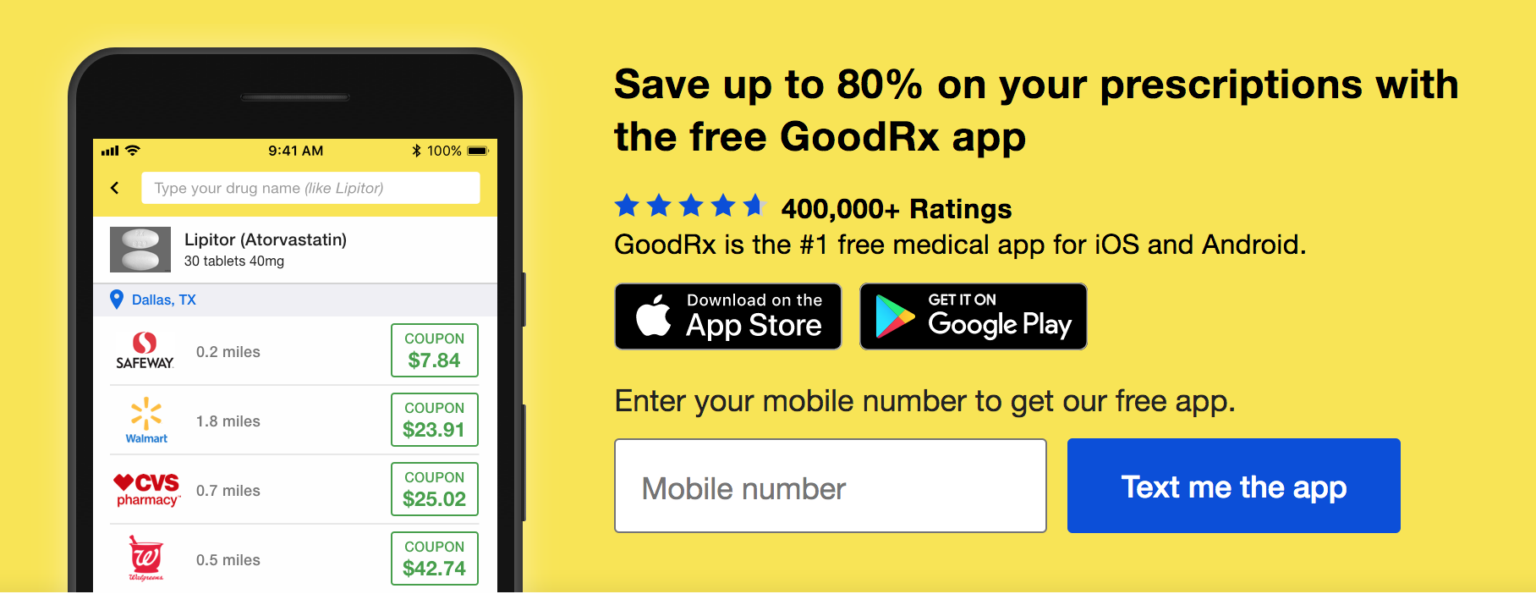Screenshot of an advertisement featuring a solid yellow background. On the left side of the image, there is a cell phone display, showcasing the user interface of an app. On the right side, in bold black letters, the advertisement states: "Save up to 80% on your prescriptions with the free GoodRx app." 

Beneath this, the app's features are described, including a rating of 4.9 stars from over 400,000 users, positioning GoodRx as the number one free medical app for both iOS and Android. There are two prominent buttons for downloading the app: one for the App Store and another for Google Play. Additionally, there's a blue box with white text urging users to enter their mobile number to receive the app via text.

The cell phone image on the left demonstrates how users can input the name of their medication into a search bar, which then displays both brand-name and generic options along with their prices. The app provides price comparisons for those without insurance, highlighting available stores where prescriptions can be filled.